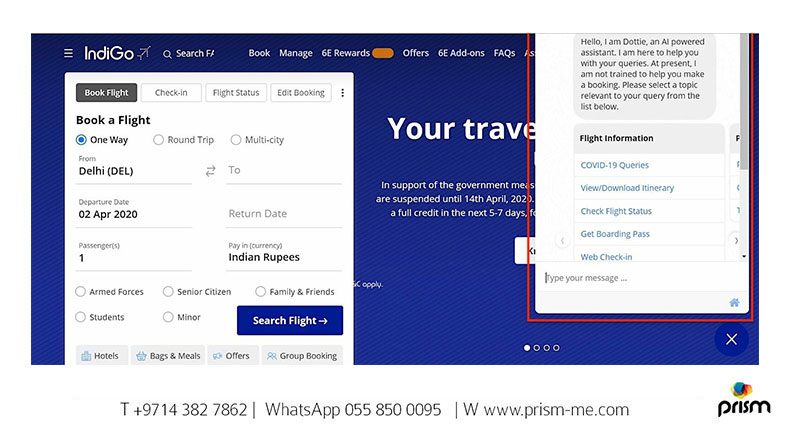The screenshot is taken from the Indigo website and illustrates its user interface. At the top left corner, there are three horizontal lines followed by the Indigo logo. Adjacent to these is a search icon. Across the top, there are several clickable options: 'Book Manage', '6E Rewards', 'Offers', '6E Add-ons', and 'FAQs'. A pop-up chat window partially obstructs the view of the interface.

Inside the pop-up window appears a message from "Dottie," an AI-powered assistant. Dottie greets the user with the message, "Hello, I am Dottie, an AI-powered assistant. I'm here to help you with your queries. At present, I am not trained to help you make a booking. Please select a topic relevant to your query from the list below." The list provides various options including 'Flight Information', 'COVID-19 Queries', 'View/Download Itinerary', 'Check Flight Status', 'Get Boarding Pass', and 'Web Check-in'. Below the list, there is a text box for the user to type in their queries.

On the left side of the page, a white sidebar offers further options such as 'Book Flight', 'Check-in', 'Flight Status', and 'Edit Booking'. The 'Book Flight' section contains sub-options for 'One-way', 'Round-trip', or 'Multi-city' flights. It also includes fields for 'From' and 'To' destinations, 'Departure Date', 'Return Date', and 'Passengers'. Additional checkboxes are available for special categories like 'Armed Forces', 'Student', 'Senior Citizen', 'Minor', and 'Family and Friends'.

At the bottom of the interface, there are tabs for 'Hotels', 'Bags and Meals', 'Offers', and 'Group Booking'. To initiate a flight search, there is a prominent blue button labeled 'Search Flight'.